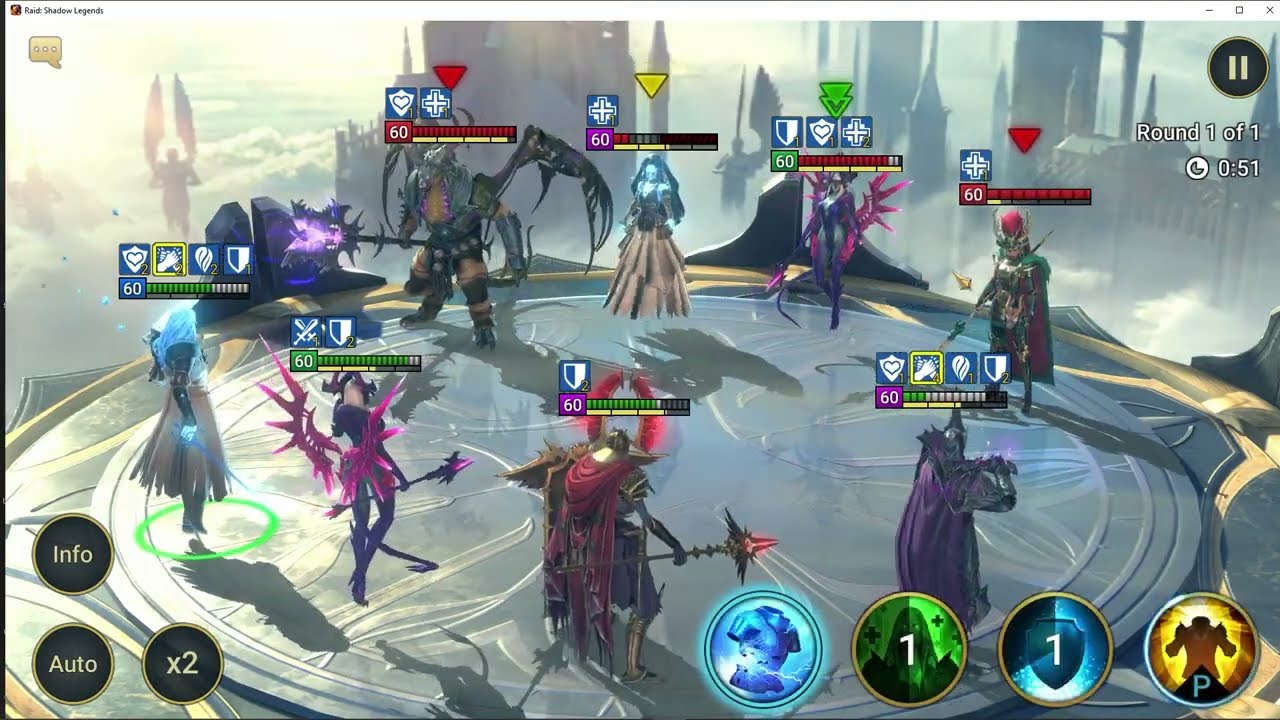This image is a highly detailed screenshot from the video game Raid Shadow Legends, likely extracted from a desktop or mobile version as indicated by the Windows minimize and close buttons in the top corner. The main focal point is a round battlefield situated in a fantasy setting, showcased with dramatic cloudy skies and grand monuments or castles in the background. On this battlefield, eight elaborately designed characters—most likely a mix of warriors, knights, and possibly a princess—are arranged in combat positions. Four characters, featuring a mixture of both male and female personas, stand on one side with health bars above them, while on the opposing side stand another four characters, some demon-like, with red health bars and various buffs and debuffs applied.

The scene is richly colored with a palette dominated by grays, blues, and golds, enhanced by sporadic touches of white, green, red, orange, purple, and yellow, adding vibrancy and complexity. In the lower right corner of the screen, there are four circular icons representing different powers or abilities available to the player, including a green circle marked with the number "1," a blue one with a "1" on a shield, and a golden symbol with the letter "P." The lower left corner features user interface buttons including "info," "auto," and a small circle indicating a 2x speed option. Additional game information is visible at the top left, where the game's name "Raid Shadow Legends" is displayed, and at the top right, indicating that the player is in "Round 1 of 1."

The overall composition and vivid details suggest a fantasy genre, immersing the viewer in an epic, strategic combat scenario within the game's universe.